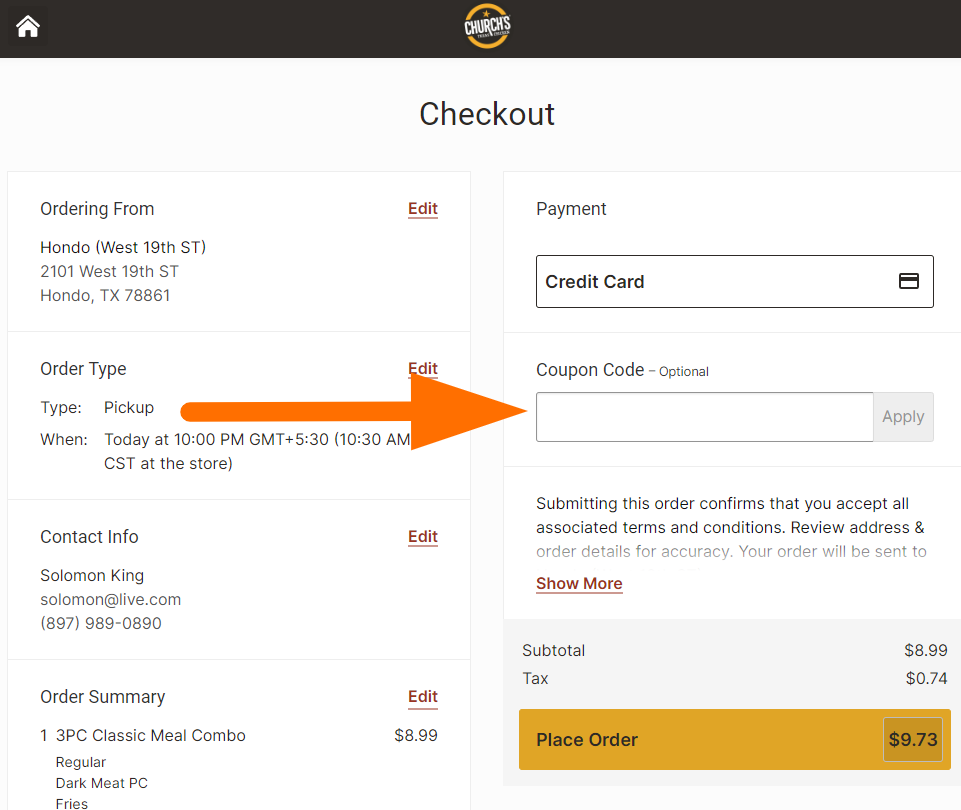This is a detailed screenshot of a mobile order interface for a Church's Chicken location. The app features prominently a logo at the top-center on a black background, comprising a yellow-orange circle with white text that reads "Church's," with a star embedded within the logo. Below the logo is a home button graphic.

The central portion of the screenshot displays the heading "Checkout" in large, bold letters. Directly beneath it, the phrase "ordering from" is written in a black font, followed by a red edit bar with a hyperlink, specifying the address: 2101 West 19th Street, Hondo, Texas, 78861. 

An orange arrow on the screen directs attention to the "order type" section, indicating "Pick Up" with an accompanying red edit hyperlink. The pick-up time is noted as "today at 10 p.m." Next to the arrow is an optional "coupon code" entry field.

The payment method shown is a credit card, accompanied by the respective logo graphic. Under "Contact Info," the details provided include the name Solomon King, with a red edit option next to it, his email address (Solomon at live.com), and his phone number (897-989-0890).

In the order summary section, it is noted that Solomon King has selected one "Three-Piece Classic Chicken Combo Meal."